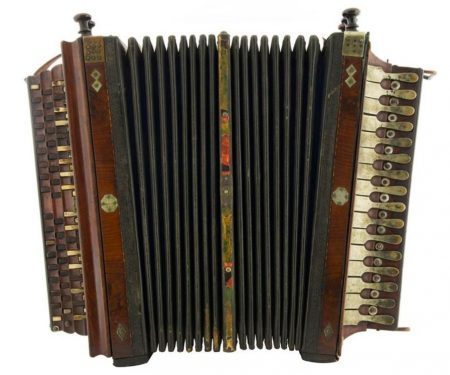The image features a vintage accordion, possibly from the 1940s or 1950s, characterized by its classic, well-worn appearance. The centerpiece of the accordion is its black bellows framed by a light gray border, which exhibits a colorful and ornate trim piece. On either side of the bellows, there are wooden panels adorned with intricate detailing, stretching vertically and capped with metallic latches, possibly in gold or silver, and decorative shapes including two diamonds and a circle at the center.

The right side of the accordion showcases piano-style keys, predominantly white, juxtaposed against metal elements, and leading down to a rectangular wooden base. These keys are notably dirty, indicative of frequent use over the decades. An array of black knobs is visible at the top of the accordion. On the left side, there are three rows of buttons, displaying a mix of gold and brown hues, also set against a wooden plate similarly an inch thick. This side is equipped for operating the air mechanism, instrumental in producing the instrument's distinctive sound. The accordion itself appears to be "floating in space" against a stark white backdrop, amplifying its aged beauty and intricate craftsmanship.